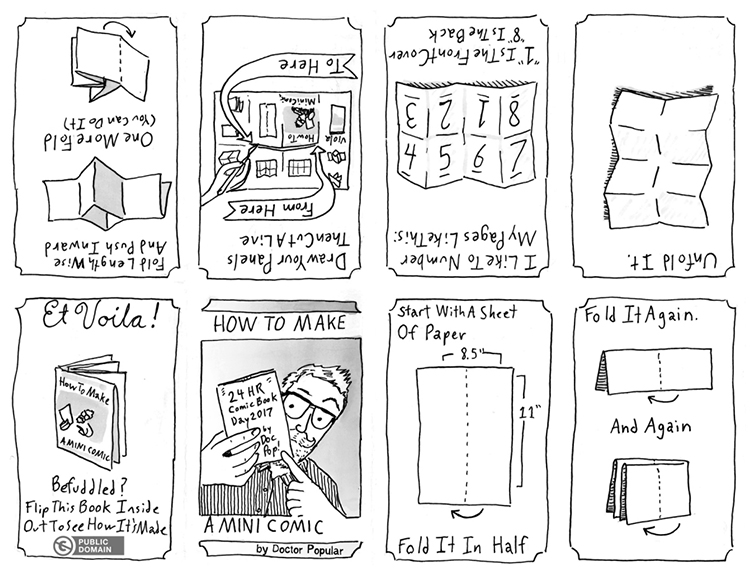This black and white image is composed of eight vertically rectangular panels arranged in a square, bordered by black lines with a white background. The top four panels are upside down, while the bottom four are right side up. The overall image provides a step-by-step guide for creating a mini-comic by Dr. Popular. The first bottom left panel reads, "Et Voila! How to make a mini-comic," followed by, "Be funneled, flip this book inside out to see how it's made." The adjacent panel features a character with a beard pointing at a book titled "24 Hour Comic Book," with the phrase "A mini-comic by Dr. Popular" beneath it.

The instructions for making the mini-comic continue across the top row, although they are displayed upside down. Starting from the top left, the first panel instructs to "fold lengthwise and push inward," then "one more fold. You can do it." The next panel to the right advises, "draw your panel then cut a line," showing detailed steps on how to do so. The third panel mentions, "I like to number my pages like this," accompanied by numbered pages. The final top row panel mentions "unfolding," indicating the next part of the process. Various simplistic, instructional drawings accompany each panel to visually guide the reader through the comic-making process.